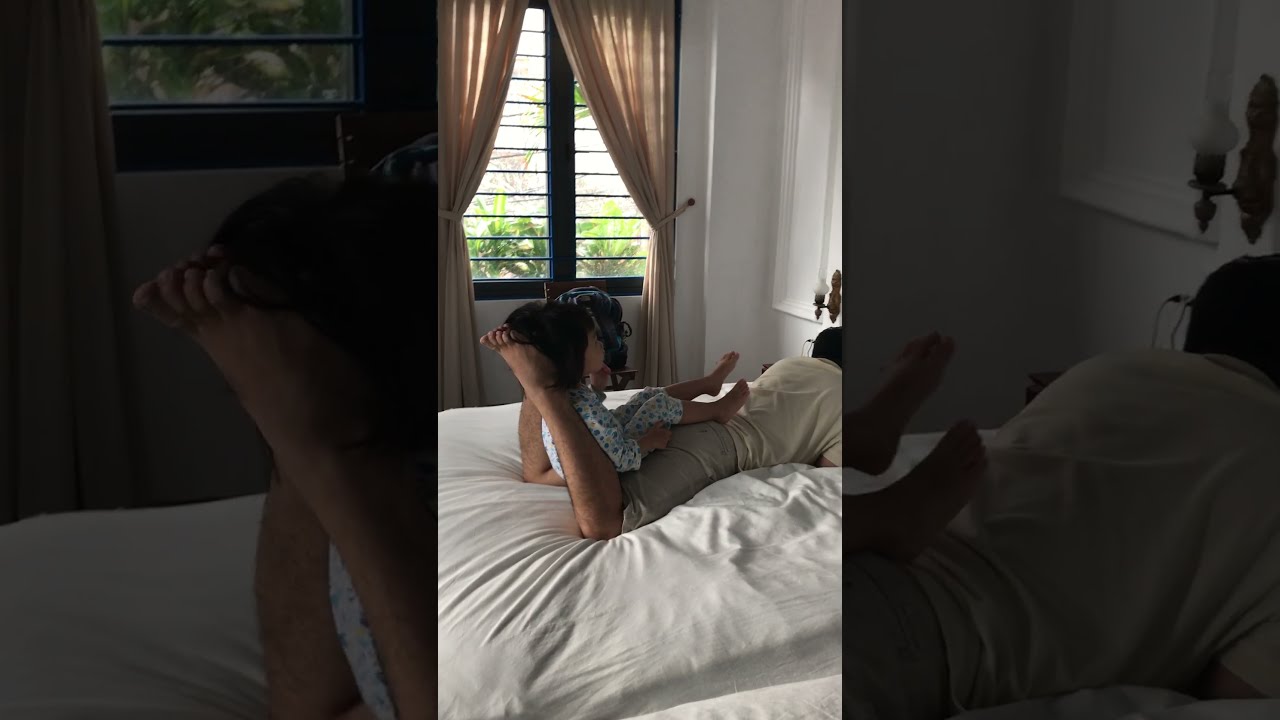A bright, sunlit bedroom with open window shades and tan curtains serves as the backdrop for a heartwarming scene. The white-walled room and white bedding create a serene atmosphere. At the center of the image, an older man lies on his stomach, his head cut off from the frame, wearing tan khaki shorts that reach his knees and a light-colored shirt. His legs are bent, forming a playful arch beneath which a young child comfortably nestles. The child's head rests against the man's feet, and her feet extend towards his lower back, exuding a sense of cozy intimacy and fun. The room is clutter-free except for a small stand in the corner holding a backpack and a light fixture mounted above the man's head, adding to the homely feel. Various colors like tan, off-white, black, green, and brown subtly punctuate the composition, emphasizing their natural and relaxed setting. The scene, devoid of any textual elements, captures a tender moment between what appears to be a father and his child during a peaceful day indoors.